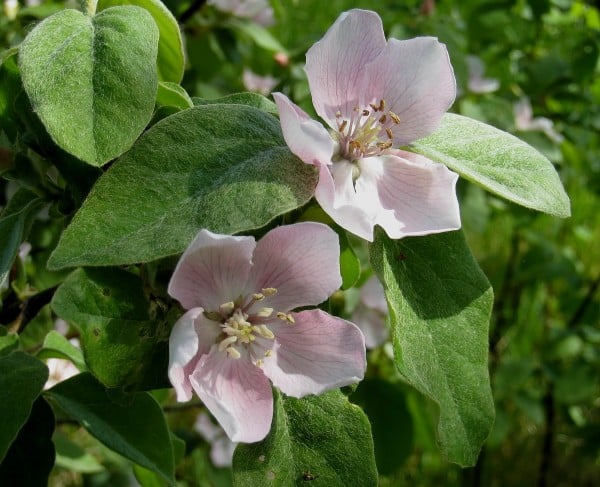This landscape-oriented photograph captures two delicate flowers in full bloom, set against a backdrop of green foliage that is softly out of focus, suggesting the use of a macro lens. The main colors in this nature image are vibrant greens and soft pinks. The flowers feature five pale pink petals that transition to nearly white at the tips, adorned with delicate, darker pinkish streaks radiating from the center. The stamens are strikingly elongated and straight, showcasing a yellowish hue with tassel-like ends that bear the pollen, adding textural detail to the image. The flowers are accompanied by large, velvety green leaves that almost rival the flowers in size, each with a prominent central vein and a pointed tip, accentuated by small white hairs that lend a fuzzy appearance. Sunlight streams in from the right side, illuminating the flowers and leaves on that side while casting the left side into shadow, creating a dynamic interplay of light and shade. The background, though blurred, hints at more leaves and flowers, enhancing the natural and tranquil ambiance of the scene. There is no accompanying text to identify the species, and no insects or other plants are visible, focusing attention entirely on the serene beauty of the flowers and leaves.